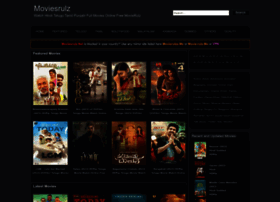The image features a dark gray, almost black background that appears blurry, especially when zoomed in. At the top of the image, there is indistinct white text that seems to read "movie rules," with a noticeable "Z" at the end. This section also includes various white words spread across it, but they are too blurry to decipher.

On the right side of the image, there appears to be a white search box accompanied by a rectangular black button with white text, possibly indicating the "search" function. A black border with similarly indistinguishable white text runs parallel to this feature.

Near the middle of the image, there is a dark gray rectangular box outlined in orange, containing multilayered text where the first two words are in red, the subsequent words are in white, followed by two words in orange. This pattern repeats with some white text interspersed, making up a complex and colorful array of information that remains unreadable due to blurriness.

Lower in the image, there's a section possibly labeled "featured," perhaps denoting "featured movies," though the exact wording is unclear. Below this heading, there are eight small, blurry images arranged in two rows, with four images in each row. These images likely represent Bollywood or Indian films, but like the rest of the text, they are too blurry to identify any specific titles or details.